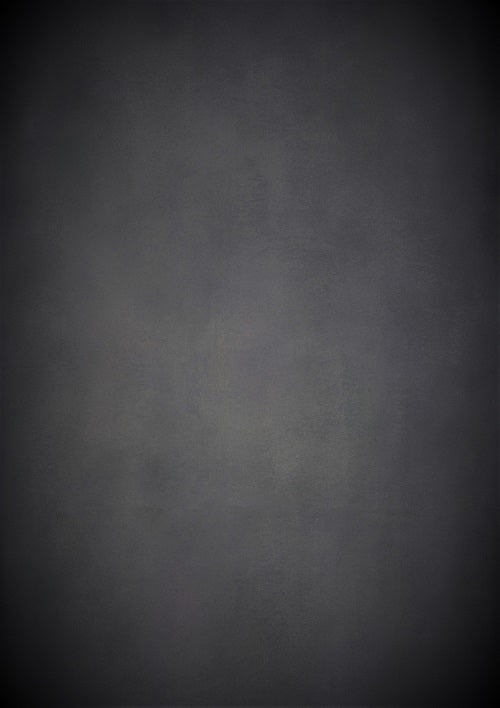The image is a vertical rectangle predominantly showcasing a gradient of gray tones. The four corners of the picture are the darkest, almost black. Toward the middle, the gray lightens slightly, with the lightest gray concentrated in the center. Sporadically, there are dark gray splotches within the lighter gray, creating subtle, indistinct shapes that some might interpret as vague facial features. The overall effect is reminiscent of a blank canvas or a minimalist background, perhaps similar to the neutral gradients used in traditional studio photography backdrops. The color palette is primarily gray, with varying degrees of black and hints of little grayish brown.